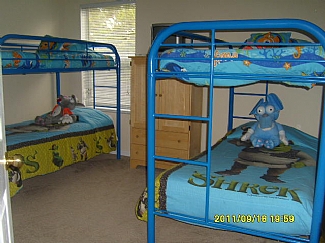This low-resolution color photograph, timestamped in yellow as 2011/09/16 at 19:59, depicts a child’s bedroom with two sets of identical blue metal bunk beds positioned within the room. The bed in the foreground on the right is neatly made with a blue Shrek-themed comforter, showing the character's name in green letters along the bottom edge. Matching yellow bedspreads hang down from the bottom bunks on both the left and right beds, adding a uniform touch. A blue anthropomorphized mouse stuffed animal sits on the lower right bed, while a grey stuffed animal with white and red accents is placed inconspicuously on the left lower bed.

The walls in the room are painted an off-white color, and a light brown carpet covers the floor. In the upper left corner of the back wall, a window with slightly open white blinds allows a glimpse of the outside. Positioned between the two bunk beds on the far wall is a beach pinewood-colored armoire, featuring two horizontal drawers at the bottom and double cabinet doors at the top. The white internal door on the left side of the image is partially visible, adorned with a brass rounded doorknob. The image is characterized by its landscape orientation, capturing the tidy and organized setup of what appears to be a child's cozy and inviting sleeping space.